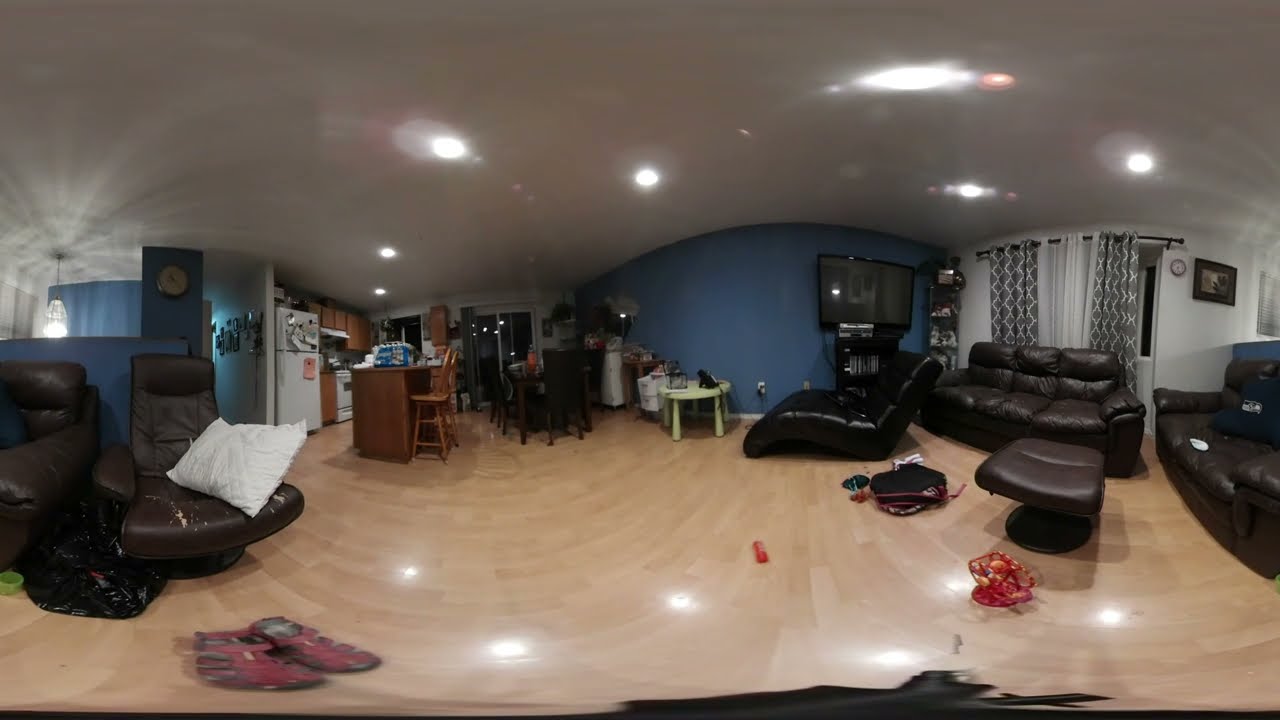The image captures an indoor scene that appears to be an apartment or living room, potentially taken with a stereoscopic 360-degree or ultra-wide lens, resulting in a warping effect. The scene encompasses three primary viewpoints in a swirling, panoramic effect. On the far left, there are two brown chairs, one with a white pillow, accompanied by a carpet in front and a lounge chair, creating a cozy and warm ambiance. Below this section is the kitchen area, identifiable by a refrigerator and a stove, and there's a dining deck nearby. Transitioning from left to right, the mid-section captures a woman, possibly a teenager, walking right to left, heading towards the left side with the pillow. This part of the image also reveals a wooden floor. The far right of the image showcases a living room setup with brown leather sofas, an ottoman, and a black chaise under a large TV mounted on a big blue wall. Additionally, there’s a window that seems to look out onto a parking lot or an exterior view. A massage chair and footrest are also visible, enhancing the comfort of the space. The ceiling features a white roof with lights reflecting off it but distorted into odd shapes due to the lens effect. Overall, the room conveys a spacious, interconnected living environment filled with various seating options, merging both kitchen and living spaces.